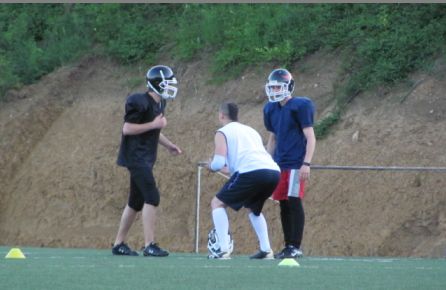The image depicts a vivid outdoor scene during a bright day on a well-lit grass field. In the foreground, two football players can be seen, both donned in their complete football gear, including helmets, and featuring a mix of dark blue, red, black, white, and gray on their uniforms. Positioned nearby is a third individual, who appears to be engaged in a workout, possibly doing squats, and notably, he is not wearing a football helmet. The backdrop reveals a dirt hill topped with patches of grass, creating a natural setting. The clarity of the photograph is enhanced by the ample natural light, contributing to a sharp and detailed depiction where colors from black to brown and from dark blue to green stand out vividly. No other individuals or vehicles are present in the frame, focusing the viewer's attention solely on the trio and their activities.